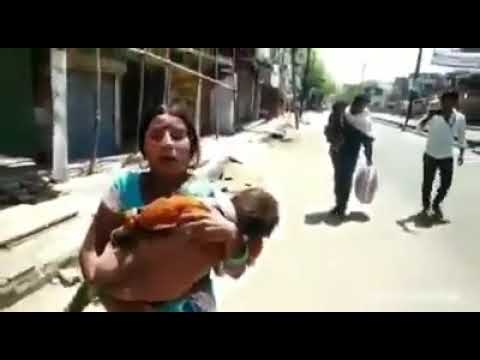In a blurry, chaotic scene, a young woman with dark black hair parted on both sides, falling just below her neck, is running down a poorly maintained, light yellow street. She has a horrified expression on her face. The woman is wearing a shirt with light green shoulders that transitions into a white color. Clutched tightly against her chest is a child with dark brown hair and an orange sleeve, with his head to her right and bottom to her left. The child appears distressed, and a bloody rag is draped over his arm.

Behind them, two men, who also appear to be of Indian descent, walk down the street. The man farthest to the right is dressed in a blue shirt and black pants, holding something on his shoulder with his raised hand. The other man wears a shirt that is white on top and black underneath, carrying a gray suitcase-like bag. The ramshackle neighborhood around them features dilapidated buildings and light poles. To the left side of the street, there is a building under construction, with stick supports and teal-colored doorways. The right side of the image shows a sidewalk and more rundown buildings in the distance. The overall setting appears to be in a distressed urban area, likely somewhere in India, capturing a grim and intense moment.